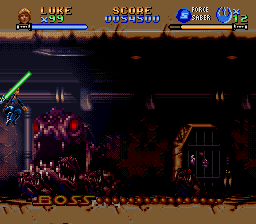This small, square, pixelated image is a screenshot from an old Star Wars video game. The top and bottom parts of the image are predominantly brown, framing a detailed scene in the center. A large, monstrous creature with red eyes, an open mouth displaying fangs, and a distinctly imposing presence dominates the middle, facing the left. Above the creature and to the left, a character identifiable as Luke is depicted mid-jump, wielding a vibrant green lightsaber. The setting has a pipe extending across the ceiling and an opening on the right, resembling a barred door or jail cell, with three figures around it. The interface displays "LukeX99" at the top left along with Luke's face and a horizontal lightsaber graphic. The score is shown centrally, reading "54,500," and to the far right, "Force Saver 12" is noted next to two icons, one gold and one blue.